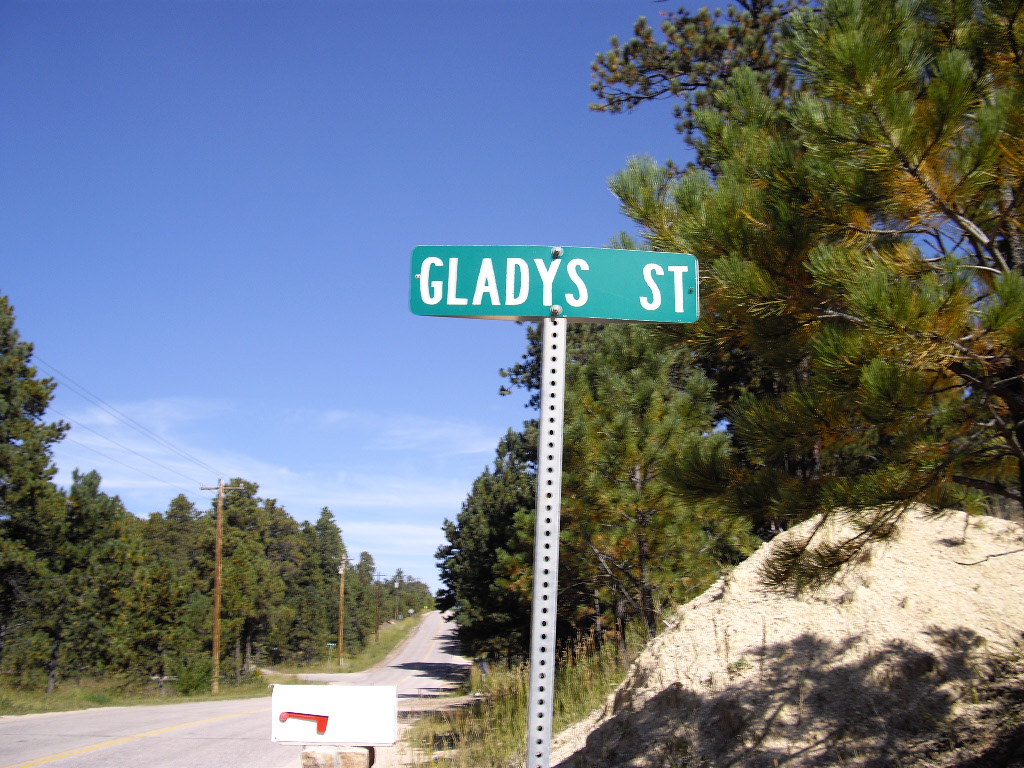This photograph offers a bird's-eye view of a serene, paved country road marked by a prominent yellow center line. Flanked on both sides by towering pine trees that stretch into the distance, the road exudes rustic tranquility. On the left side, the trees give way to a lush patch of grass, adding to the rural charm. The right side of the road mirrors this natural setup but also features a mailbox standing as a humble sentinel. Dominating the center of the image is a metal pole adorned with a classic green street sign reading "GLADYS" in bold white letters. Below the dense branches of the pine tree on the right sits a large, weathered rock, its surface dappled with shadows cast by the foliage above. A series of telephone poles and wires run parallel to the road, adding a touch of infrastructure to the otherwise untouched landscape.